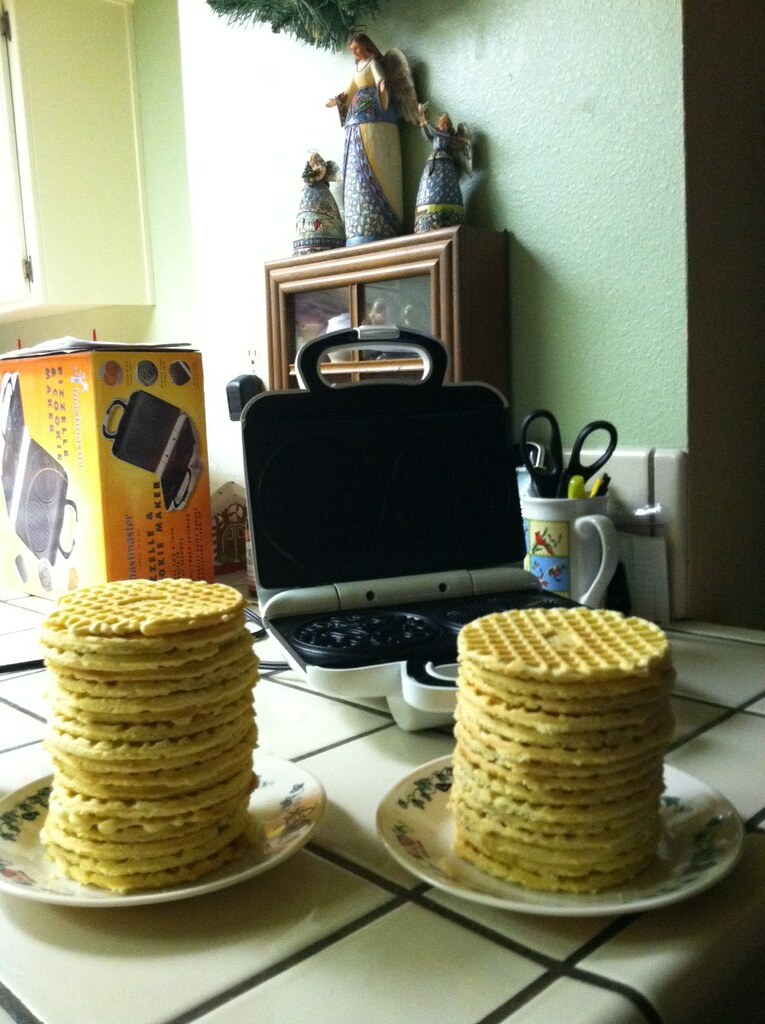This detailed photograph captures a vibrant kitchen scene centered around a bountiful breakfast spread. In the foreground, two ceramic plates adorned with a delicate floral border are each piled high with stacks of thin, circular waffles, golden yellow in color, with each stack containing over a dozen waffles. These plates rest on a white tiled countertop with contrasting black mortar lines. Just behind the plates, there's an open waffle maker with a white exterior and black interior, exhibiting its functional cooking plates and handle. To the left of the waffle maker is an orange and yellow box featuring an image and text detailing the same appliance. A white ceramic mug with colorful illustrations, including red, blue, and a yellow backdrop, holds a pair of black scissors and several markers. This assembly is set against a mint green wall, with a wooden cabinet in the background, topped with ornate ceramic figures in white and blue, providing an elegant touch to the setting.